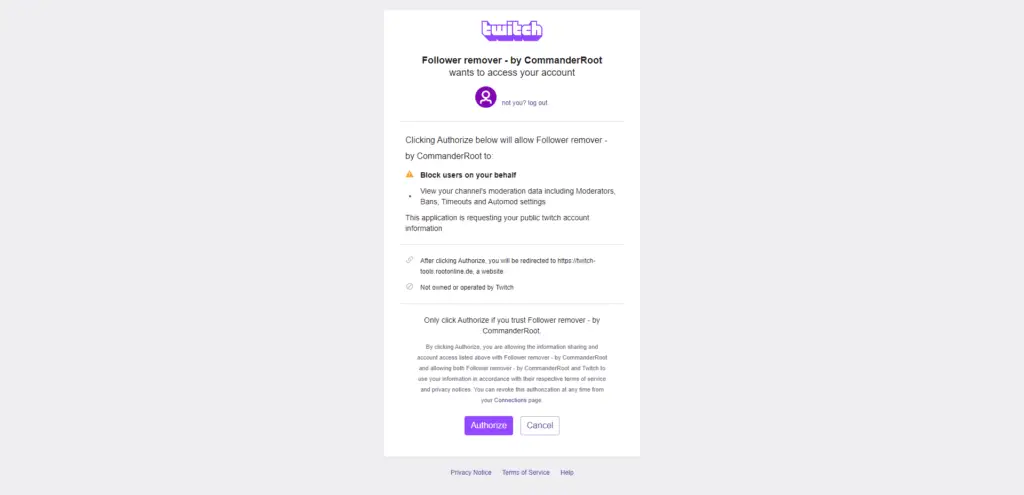A screenshot of a cell phone displaying the Twitch website authorization page for "Follower Remover" by CommanderRoot. At the top of the screen, "Twitch" is prominently displayed in bold purple letters against a vertical white rectangle background. The page requests account access, indicated by the text "Follower Remover by CommanderRoot wants to access your account" in gray. Below, a purple circle with a white person silhouette appears alongside the prompt "Not you? Log out" in gray.

Further down, instructions in bold black letters beside a yellow triangle icon explain, "Clicking 'Authorize' below will allow Follower Remover by CommanderRoot to:" followed by a bullet point detailing permissions: "View your channel's moderation data including moderators, bans, timeouts, and AutoMod settings." The application specifies it is requesting public Twitch account information, all displayed in gray.

A paperclip icon precedes the note, "After clicking 'Authorize,' you will be redirected to https://twitch-tools.rootonline.de, a website not owned or operated by Twitch," in gray. A warning circle icon with a horizontal slash emphasizes this disclaimer. The guidance concludes, "Only click 'Authorize' if you trust Follower Remover by CommanderRoot," followed by terms of service and privacy notice details in gray about information sharing and account access.

At the bottom left, a prominent purple button labeled "Authorize" in light purple invites the user to proceed, with a white "Cancel" button in gray to its right.